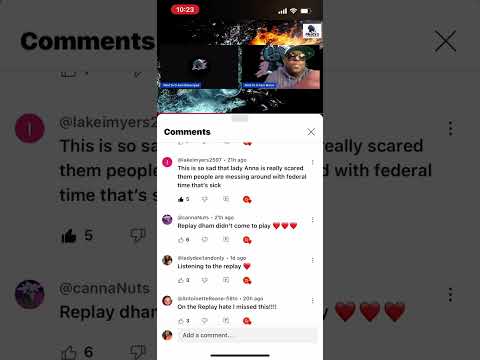In the background of the image, the word "comments" is clearly visible within a grayed-out area. Accompanying this, there's a notable red circle with a letter inside it, alongside a person's name, "At Lake I Am Yours." A snippet of their text reads, "This is so sad." The words "scared" and "with federal time" are also discernible before the text ends. This particular comment has garnered five likes. 

Adjacent to this comment is another profile image along with the username "Canna Nuts" and the word "replay," followed by three heart icons. 

Central to the image is a vertical rectangle displaying the time "10:23" encased within a red circle. Below this timestamp are several profile pictures, including one of a man wearing a hoodie and sunglasses. Surrounding these are black boxes, one of which, in the upper right corner, appears to contain an image of fire. 

Further into the comments section, the repetitive word "comments" reappears, as well as some previously illegible comments which are now readable. Among these are remarks expressing sadness and concern, stating, "This is so sad" from "Lady Anno" and mentioning, "People are messing around with federal time, that's sick." These comments are similarly marked with hearts and likes underneath them.